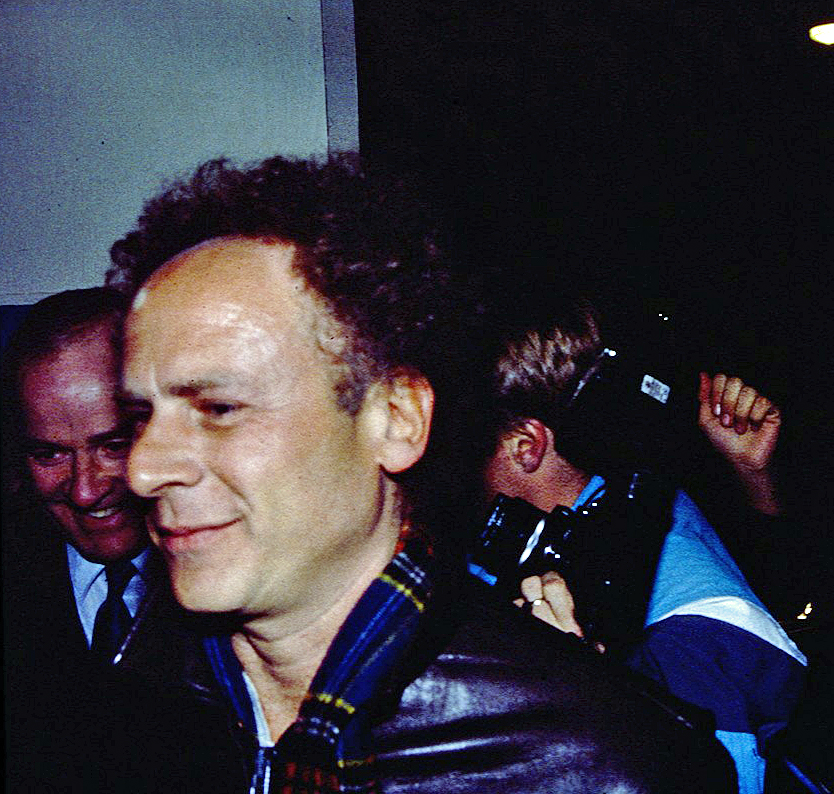The photograph captures a close-up image of a middle-aged or older Caucasian man with short curly dark hair that is thicker at the back and a slightly chunky nose. He has fair, pale skin and is smiling subtly while facing slightly to the left. He is wearing a dark jacket over a white shirt with a multi-colored plaid scarf of blue, yellow, and red wrapped around his neck. The grainy texture of the image gives it a nostalgic, older feel, reminiscent of the 70s or 80s.

In the background, to the left, there is an older man wearing a dark suit and a light blue shirt with a black tie, his face appearing red due to the photograph's artifact. To the right, another man is visible, dressed in a blue and white windbreaker, holding a professional camera up to his face. Additionally, there is a raised fist visible to his right. The background features a white and gray wall on the left half, transitioning to plain black on the right, with a ceiling light faintly seen.